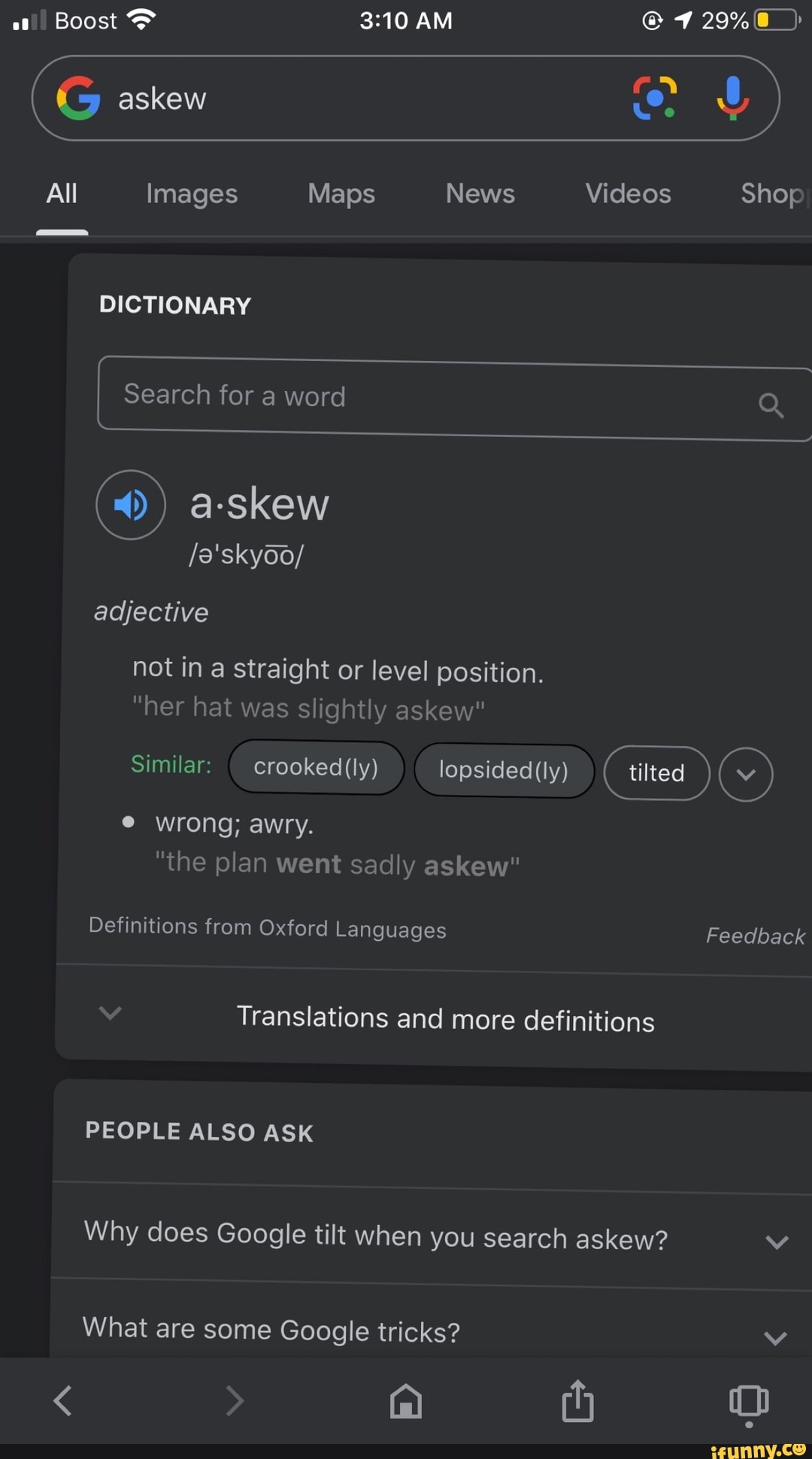The image is a detailed screenshot from a mobile device captured at 3:10 a.m. The device is connected to Boost Mobile with two signal bars and full Wi-Fi strength. The lock screen and location services are enabled, and the battery life is at 29 percent, indicated by a yellow battery icon. 

At the top of the screen is the Google logo in its iconic red, yellow, green, and blue colors. In the Google search bar, the word "Askew" (A-S-K-E-W) has been typed. Below, the device displays the search results under the "All" tab, including the dictionary definition. Other tabs visible are Images, Maps, News, Videos, and Shopping.

The dictionary section shows the word "Askew" with a pronunciation icon. The definition is provided as "adjective: not in a straight or level position," exemplified by the sentence "Her hat was slightly askew." Additionally, the Google camera logo and microphone icon are visible within the search bar.